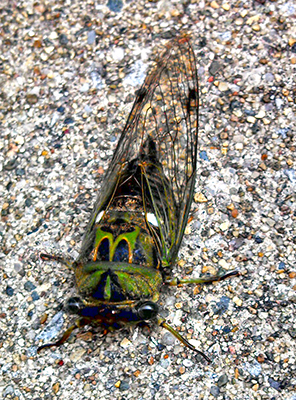The image depicts a detailed close-up of a cicada perched on a stone surface composed of tiny, colorful pebbles. The cicada, predominantly green with a shimmering rainbow effect on its head, showcases a striking contrast against the pebbly backdrop. Its transparent wings reveal the intricate pebble texture below. With six legs spread out symmetrically, two front legs angle forward while the other four splay out horizontally. The image, taken from an overhead perspective, is bright, clear, and filled with natural lighting, accentuating the intricate details and vivid colors, including subtle hues of black and orange on the cicada’s body. This vibrant setting, free of any text or additional elements, centers solely on the cicada and its fascinating features, capturing the essence of this lone insect in a clear, high-resolution photograph.